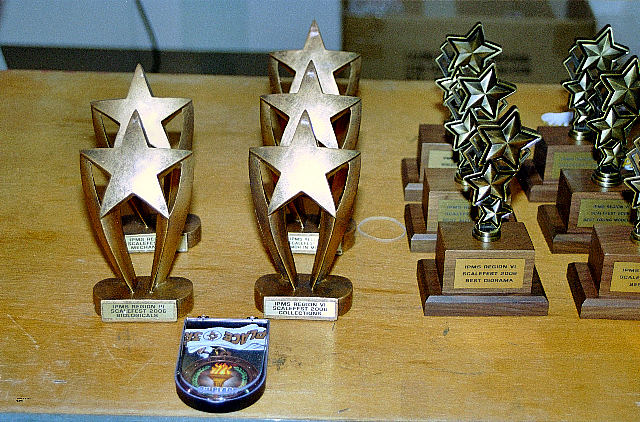The color photo features a light brown wooden table background, weathered with nicks and scrapes, and even a beige rubber band in the center. Resting on the table is a collection of trophies arranged in four rows. To the left, two golden star trophies on a wooden base form the first row, followed next by another three identical trophies. The subsequent rows have trophies on a rectangular wooden base topped with a splay of smaller bronze stars, each row containing three trophies of varying sizes. Some scratches on the table, especially on the left-hand side, show distinct black and white marks. The details on the trophies are not clear, but letters are visible upon closer inspection.